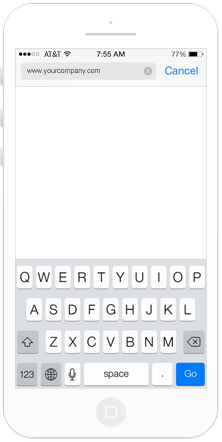This image depicts a smartphone screen resembling a text messaging interface. The device appears to be an iPhone, displaying multiple interface elements succinctly detailed. At the top-left corner of the screen, within the phone's status bar, there are three buttons. Above the screen, five small indicator dots are visible—three of which are filled in while the remaining two are blank, possibly representing signal strength indicators or other status indicators.

On the screen's top row, the carrier is labeled as "AT&T" next to an active Wi-Fi signal icon. Displayed on the upper-right is the time marked as 7:55 a.m., adjacent to a battery icon indicating 78% charge remaining.

Directly beneath the status bar, a gray border runs along the top with the text "www.yourcompany.com" on the left and a blue "Cancel" button on the right. Below this border lies the main screen area, represented by a large white rectangle.

The virtual QWERTY keyboard is displayed at the bottom section of the screen, comprised of three rows of keys. The third row uniquely includes an up arrow (shift key) on the left and a backspace button on the far right. Directly beneath this keyboard are additional function keys including a microphone icon, a space bar, a period key, and a blue "Go" button situated in the bottom-right corner.

Finally, at the bottom-center exterior of the phone is the recognizably gray circular Home button featuring a square icon in the middle, further affirming the device as an iPhone model.